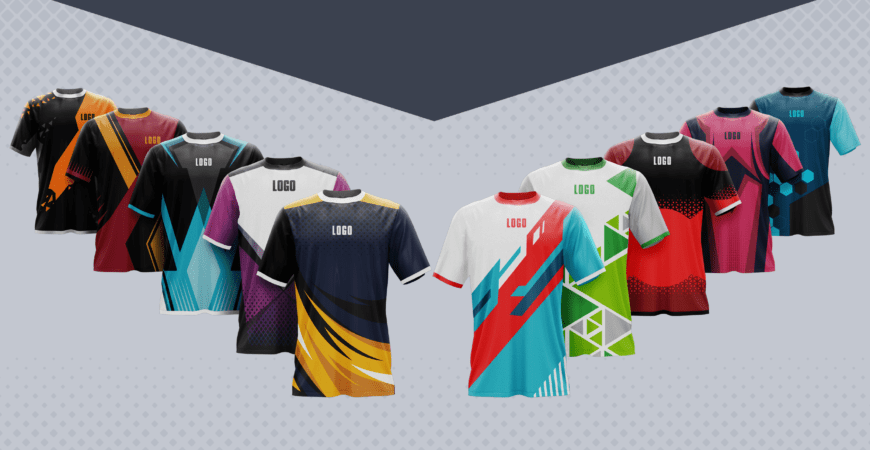The image showcases a computer-generated mock-up of 10 short-sleeved sports jerseys arranged in a wide V-shape. The jerseys are symmetrically displayed in two diagonal rows extending from the center: one row rises towards the left and the other towards the right. Each jersey features a centered "logo" text, indicating placeholders for customizable logos. The jerseys are vibrantly colored, featuring combinations such as black-orange, black-red-yellow, black-medium blue-light blue, light purple-dark purple-white, navy blue-black-yellow-white, white-medium blue-red, white-gray-green, red-black-maroon, red-black, and medium blue-light blue-black. The background is a gradient of light gray to dark gray, with a black triangle at the top, framing the display.